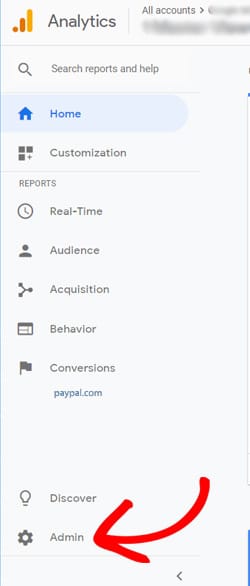This image appears to be a partially obscured and unclear screenshot, likely from an analytical or financial dashboard. At the top of the screen, a navigation bar displays options such as "Analytics" and "All Accounts," though these elements are somewhat faded, potentially indicating confidential information. Additional navigation options include "Search," "Reports," and "Help." 

Prominently featured is a section for "Reports," listing categories like "Real-Time," "Audience," "Acquisition," "Behavior," and "Conversions." A reference to "paypal.com" suggests that a PayPal account is linked to this dashboard, reinforcing the likelihood that this is a financial or e-commerce analytics tool. 

Also visible are other navigation elements labeled "Home" (highlighted in blue and accompanied by a home icon), "Customization," "Discover," and "Admin." At the very bottom, the "Discover" and "Administration" tabs are seen along with a notable red arrow pointing towards the "Admin" section, indicating a possible focus or recommendation for action in that area. Overall, the screenshot seems to be of a financial analytics interface, monitoring various aspects of account activities and reports.